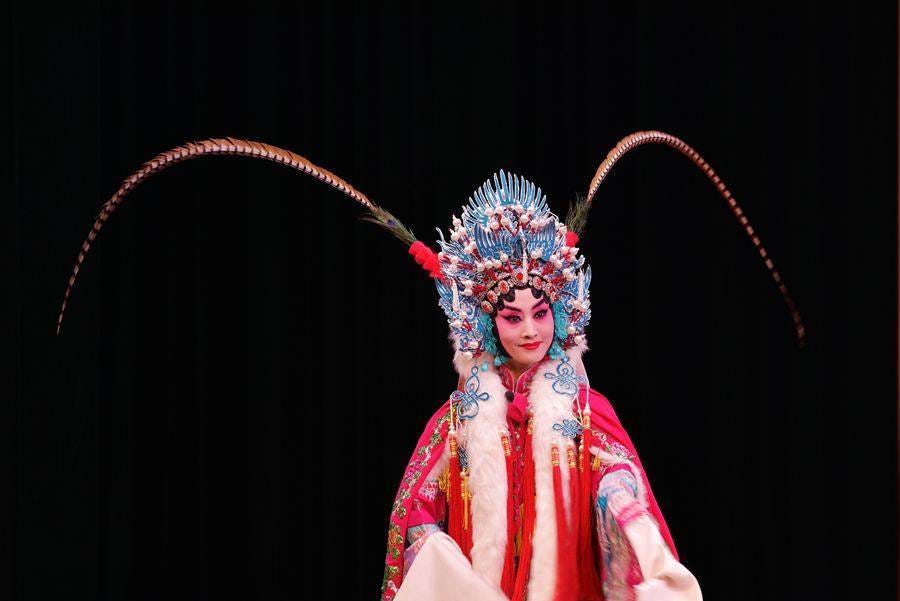The image captures a striking woman set against a black background, adorned in elaborate attire. Her face is heavily made up with almost white foundation, stark red around the eyes, and dark, defined eyebrows. Her lips are painted bright red, and she gazes intently at the viewer, her head tilted slightly to the side. She wears an elaborate crown made of shiny blue pieces and shells, from which extend two feather-like "antennas" over each shoulder. Her outfit includes a hot pink gown or cape with a white, fuzzy trim on the front. Blue earrings dangle from her ears, complementing the ornate crown. Additionally, green grasses or similar adornments sprout from the crown on her head. The vivid colors of her attire and headgear contrast sharply with the dark background, suggesting a performance or staged event, although the exact nature remains undefined.